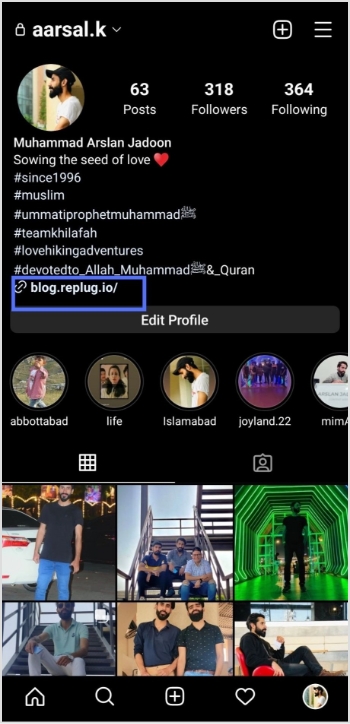This vertical image appears to be a screenshot of a social media profile, likely Instagram, accessed via someone's smartphone device. The background is uniformly black, offering no texture or dimension. 

In the top left corner, there's a small padlock icon followed by the username "arsal.kaarsal.k." On the right side, there's a plus sign icon and three horizontal lines indicating more options.

Below is the user’s profile picture encased in a circle, accompanied by some account statistics: 63 posts, 318 followers, and 364 following. The profile name "Muhammad Arjan Jadoon" is displayed prominently, followed by the bio: "Sowing the seed of love" with a heart icon. The bio also includes several hashtags: #since1996, #Muslim, #UmadiProphetMuhammad, #teamKhilafah, #lovehikingadventures, #devotedtoAllahMuhammadandQuran.

A blue box surrounds the link "blog.replug.io/edit profile," indicating an editable profile section. This box also highlights some circles representing friends or connections that one can click on. 

Below this section, a grid and a person icon suggest navigation options for viewing the user's posts and tagged photos. Following this, thumbnails of the user's posted images are displayed.

Finally, the bottom of the screenshot features familiar icons for home, search, create (plus sign), activity (heart), and profile navigation.